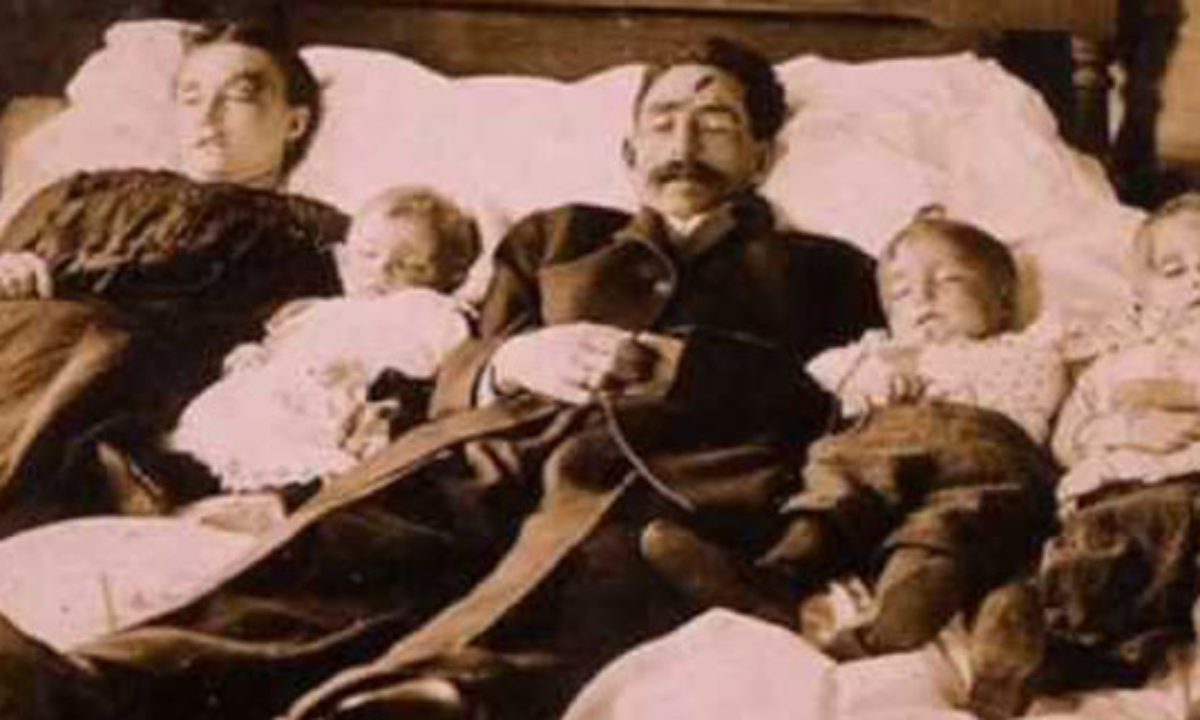The photograph appears to be an old, slightly out-of-focus, sepia-toned image capturing a family lying in bed. The scene is somber and possibly indicative of either sleep or death. Positioned on a white bedspread with a dark oak headboard behind them, the mother lies on the far left wearing a black dress with a visible bruise above her right eye. Next to her is a baby in a white lacy dress and dark shoes. The father, centrally placed, is dressed in a dark suit and has a prominent mustache. His hands are folded over his stomach, possibly holding a pocket watch, and he bears a dark mark or potential wound on his forehead. To the father's right, two children lie close by: both in light tops and dark trousers, with their eyes closed. The child on the far right is slightly cut off. Their overall appearance, along with the parents', suggests they might have sustained injuries, adding to the eerie and antiquated feel of the photograph.